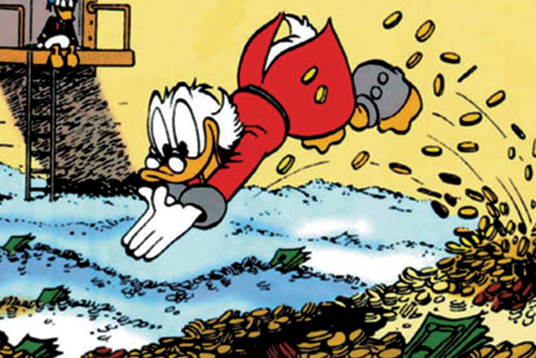The animated image portrays Scrooge McDuck, a character known from the Daffy Duck cartoons, in the midst of an exuberant dive into a massive pile of money. Dressed in his trademark red coat with gray wrist cuffs, tiny glasses perched on his beak, and gray shoes that only cover his heels, Scrooge is depicted smiling widely in mid-air, hands positioned in a traditional dive pose. Surrounding him, the foreground is filled with scattered yellow coins, transitioning into a bluish hue as they extend further back, intermingled with green dollar bills. The background showcases a yellowish wall and what appears to be grassy terrain adjacent to the immense heap of gold coins. On this grassy area, there are small clusters of dollar bills protruding, suggesting a lush landscape of wealth. A notable feature in the backdrop is a large tree trunk with a wooden platform attached, accessible by a ladder. This platform serves as a vantage point for a smaller, darker duck character, possibly wearing a dark shirt, who observes Scrooge McDuck's joyful dive, much like a lifeguard overseeing a bustling swimming pool.